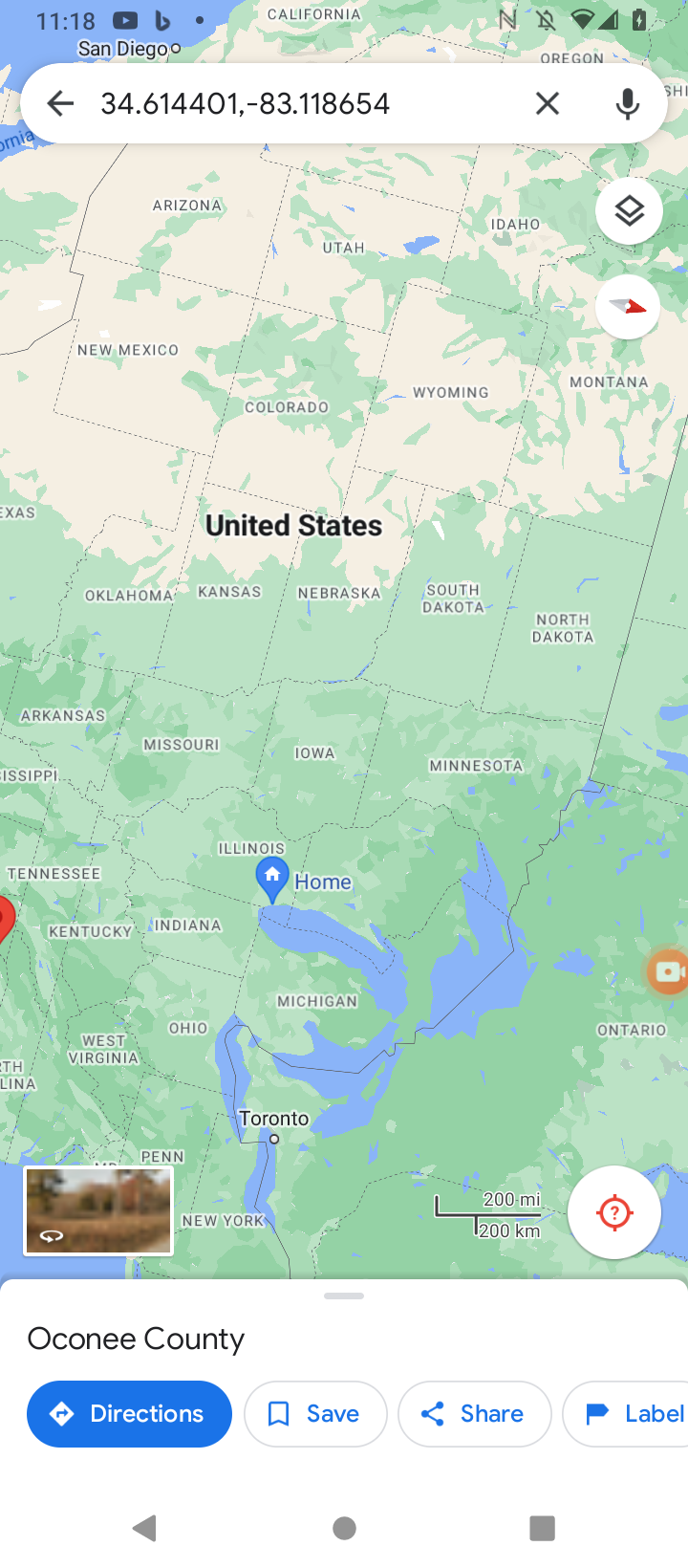A detailed caption for the image could be:

"A rotated screenshot of Google Maps centered on the United States. The map is oriented with California at the top, New York at the bottom, and Texas to the left, presenting a flipped perspective. The coordinates '34.614401, -83.118654' are entered in the search bar, suggesting a specific location search. The word 'United States' is prominently displayed in the center of the map. The bottom of the screenshot indicates the region 'Oconee County.' This screenshot appears to be taken from a smartphone, reflecting typical mobile interface elements."